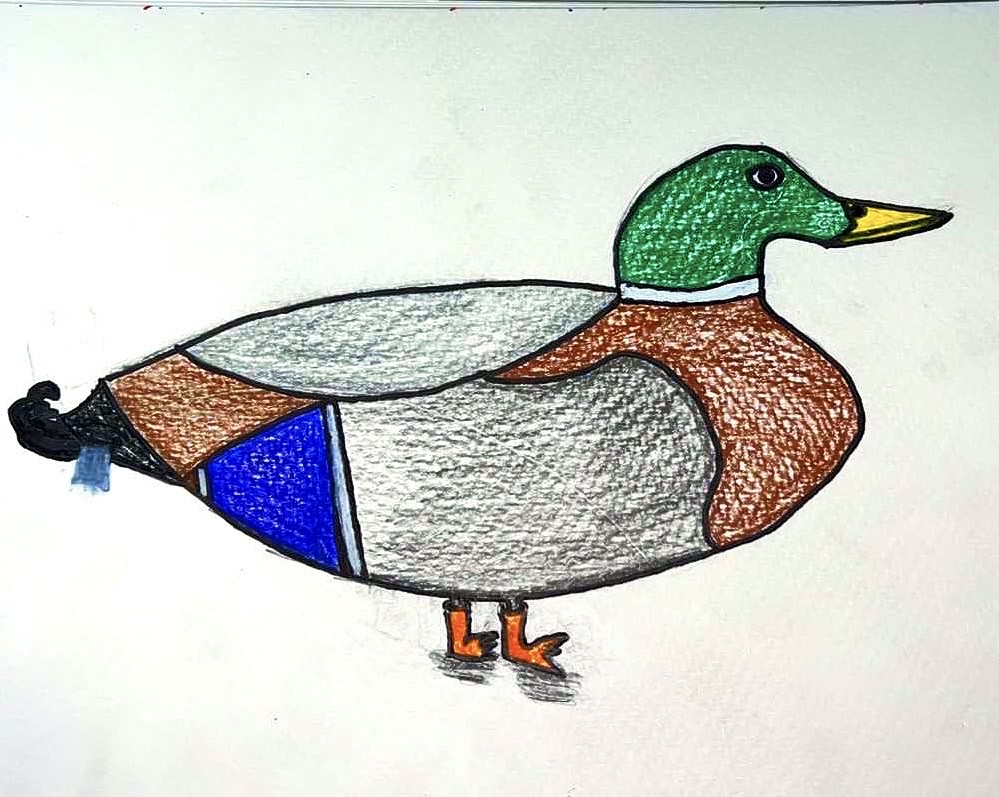This is a detailed drawing of a mallard duck, expertly colored using either crayon or colored pencils. The artwork features a black outline that delineates the distinct sections of the duck. The mallard has vibrant orange feet and a bright yellow beak. Its head is a striking green, accented by a white band around its neck. The duck's breast is a rich brown, matching some of the hues on its tail, while the belly and back are colored in shades of gray. Adding to its picturesque appearance, there is a patch of royal blue on the side, and the tips of the tail feathers are black, curling slightly upwards. This profile view of the mallard is set against a backdrop of white paper, creating stark contrasts. Additionally, a shadow is carefully etched beneath the duck, adding depth to the image.